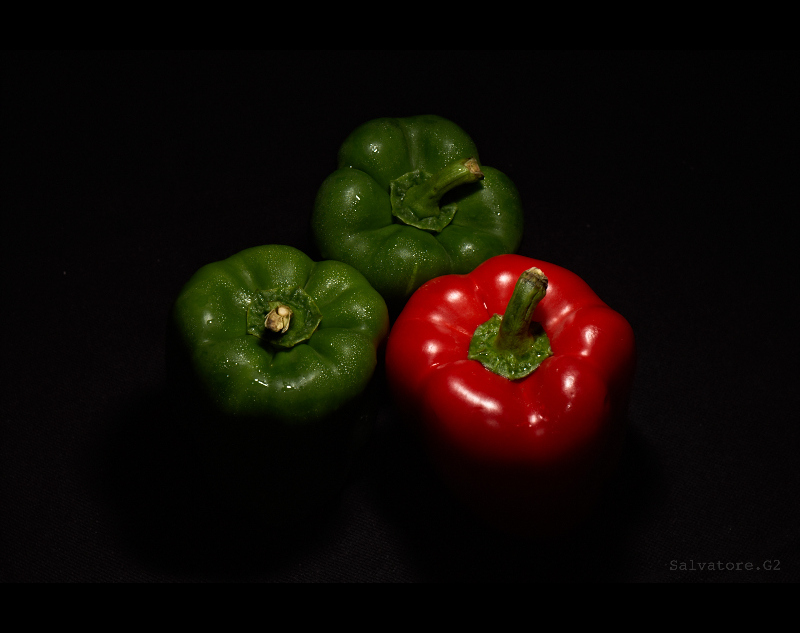In the photograph, three fully intact, fresh-looking bell peppers are prominently displayed against a completely dark background. The trio, arranged in a triangular shape, consists of two green bell peppers and one larger red bell pepper. Each pepper has a visible green stem, contributing to their freshly-picked appearance. The peppers are glistening under the direct light, highlighting tiny water droplets that suggest they were recently washed. The reflection of the light off their smooth skins further emphasizes their freshness. The image includes a watermark at the bottom right corner that reads "Salvatore.G2." The overall composition captures the vibrant colors and textures of the peppers, making them appear larger than average and very appealing.